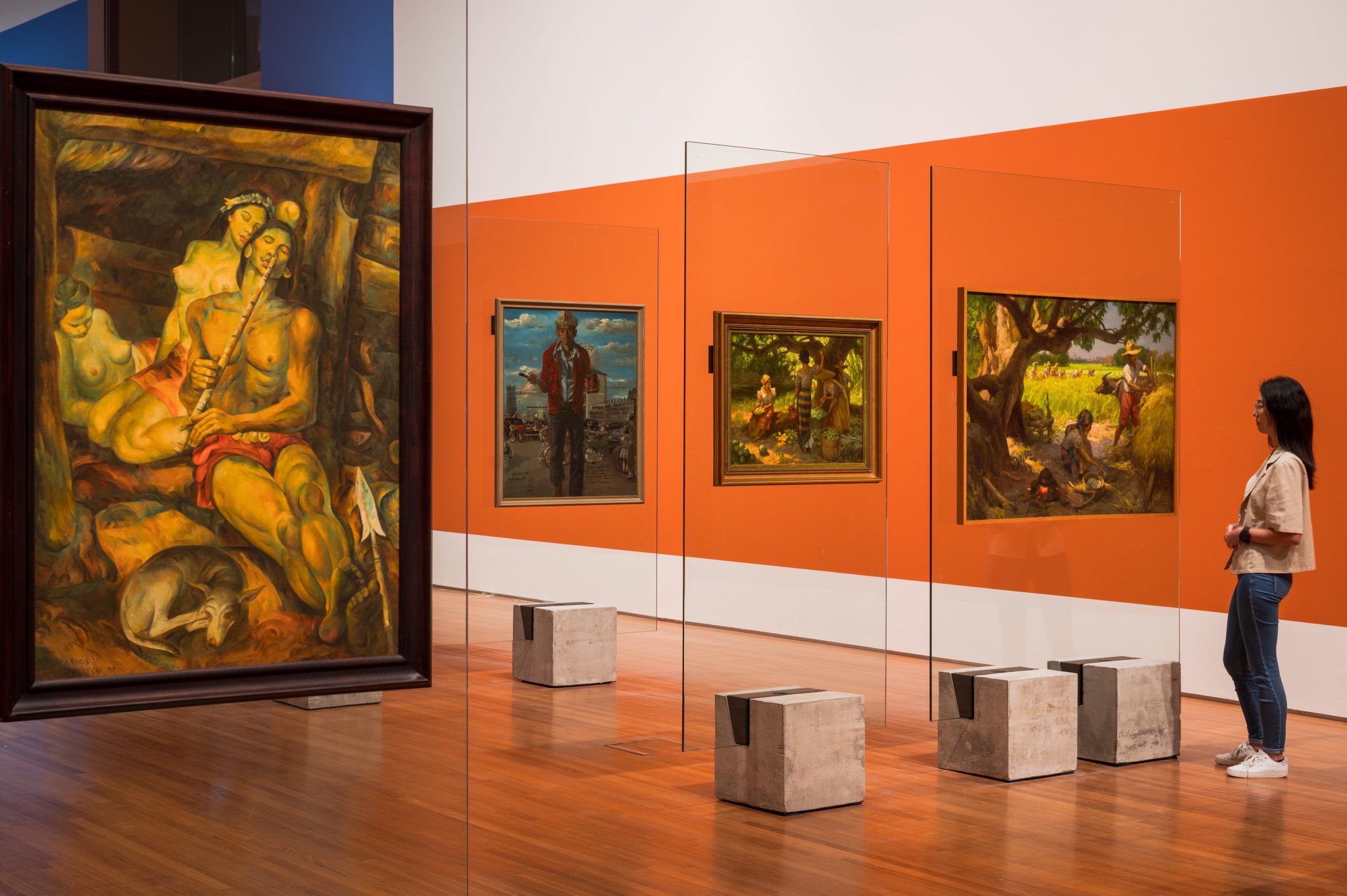This rectangular photograph depicts an art gallery room, wider than it is tall, featuring vibrant walls and a shiny wood floor. On the right side, we see a woman with long black hair, wearing blue jeans, white tennis shoes, and a beige top. She is intently observing a row of paintings held up by cut cinder blocks supporting clear glass panes. The wall she faces has an orange border at the bottom, transitioning to white above and punctuated by a prominent orange rectangle, with blue visible behind the large painting on the left. 

The foremost painting depicts a serene scene with a farmer and farmhand harvesting crops in a green field under a cyan sky. Highlighting brown-based, green-leaved curled trees, the image portrays additional, yet indistinct, workers in the background. Adjacent to this is a smaller painting illustrating a woman in a yellow and black striped dress talking to another woman in an orange-red dress. Both are amidst a sunny clearing with baskets of fruits or vegetables. Further back, a third painting shows a man in a red vest, cyan undershirt, and dark pants, standing against a cyan sky with indistinct background elements, including a vehicle and a silo.

Dominating the left side, a large painting in a wooden frame captures a scene of two nude women and a shirtless man holding a flute upright. The man, in red shorts, is accompanied by a dog and shares the cabin setting with the women, one of whom has a headband. The tonal variations in the cabin’s brown walls and the dog’s beige face and legs contrast sharply with the vivid shorts worn by the figures. The cohesive yet diverse visual elements enhance the gallery’s artistic narrative, balancing large and small paintings, traditional and whimsical elements, all under a calm, ambient light reflecting off the pristine wood flooring.